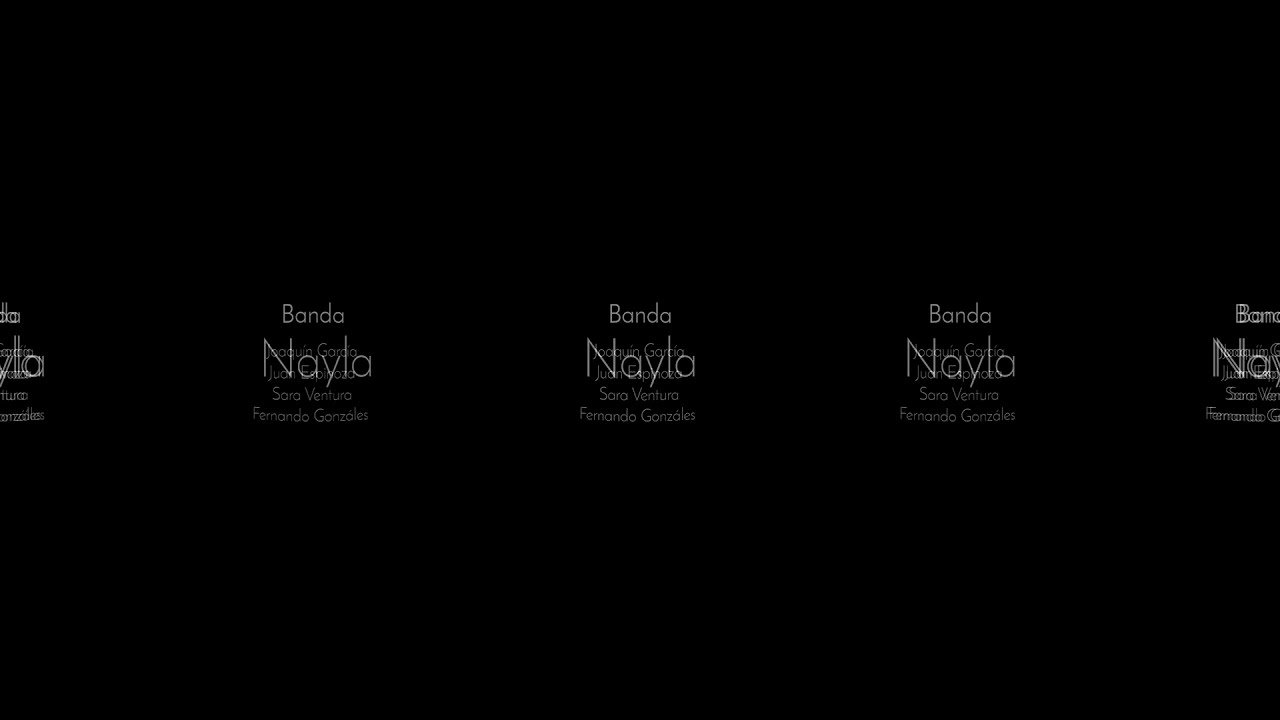The photograph features a rectangular image with a black background, prominently displaying repeating text in the center. The repeating text consists of the word "Banda" in small white font, followed by the names "Joaquin Garcia," "Juan Espinettio," "Sara Ventura," and "Fernando Gonzalez" in a sans-serif font. The first two names, "Joaquin Garcia" and "Juan Espinettio," are partially obscured by the larger word "Naila," which is written in an elegant, larger white font, adding a classy touch to the image. This sequence repeats five times horizontally across the center of the image, with the furthest left and right instances partially cropped out. The overall effect is a sophisticated watermark-like logo pattern that stands out against the dark background.